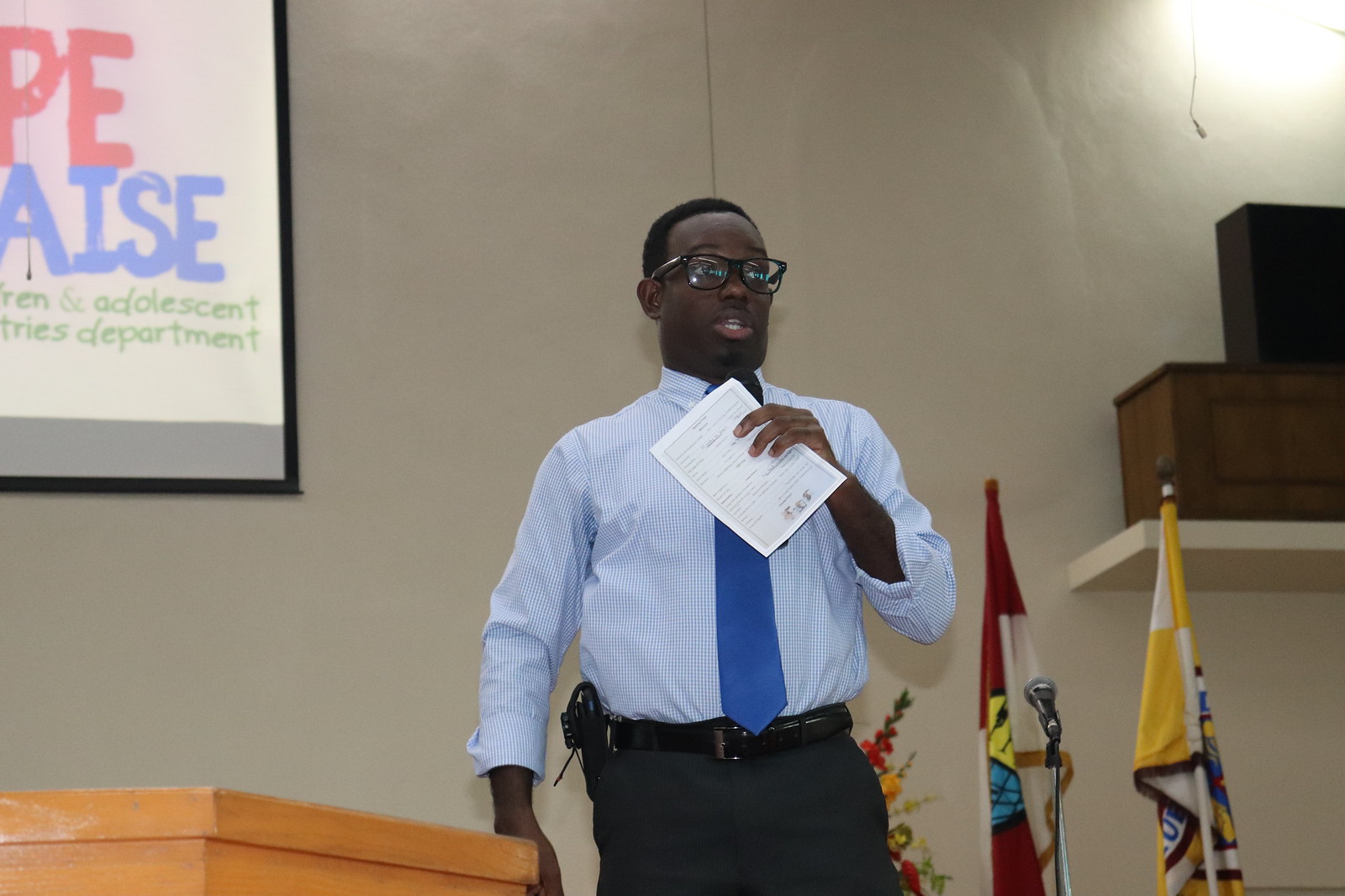A black man is captured mid-sentence while standing at a podium, addressing a crowd. He is dressed in a blue dress shirt, blue tie, and dark slacks, complemented by black glasses. In his left hand, he holds a piece of paper with writing on it. Behind him, a white wall features a partially visible slide presentation in the top left corner. To his right, there are two small flags and a forward-facing microphone, with speakers positioned above them. A shelf on his left holds two boxes, and he appears to have a radio or similar device on his belt, adding further context to his role, possibly as a city council politician or speaker.